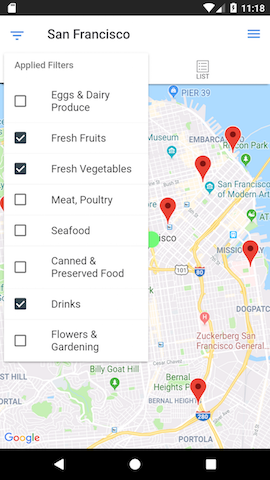The image on the cell phone screen displays several elements in detail. At the top, in a black bar, the time is shown as 11:18 in the top right corner, alongside a fully charged battery icon and good cellular connection indicators. There is also a lock icon on the left side of this black bar. The text "San Francisco" is displayed slightly off-center to the left.

Below the black bar, the screen features a blue icon of a triangle with lines to the left and a box with lines to the right, labeled "Applied Filters." 

An overlay pop-up box lists several categories: "Eggs and Dairy," "Produce," "Fresh Fruits," "Fresh Vegetables," "Meat, Poultry, Seafood," "Canned and Preserved Food," "Drinks," and "Flowering and Gardening." The categories "Fresh Fruits," "Fresh Vegetables," and "Drinks" are checked off.

The white box overlaying the map contains location pins in red, which denote the locations relevant to the selected categories. The map includes details such as interstates, side streets, a pier, and areas of water and land. The water is depicted in blue while the land is shown in white.

Below this map are small, typical smartphone icons positioned neatly at the bottom of the screen.